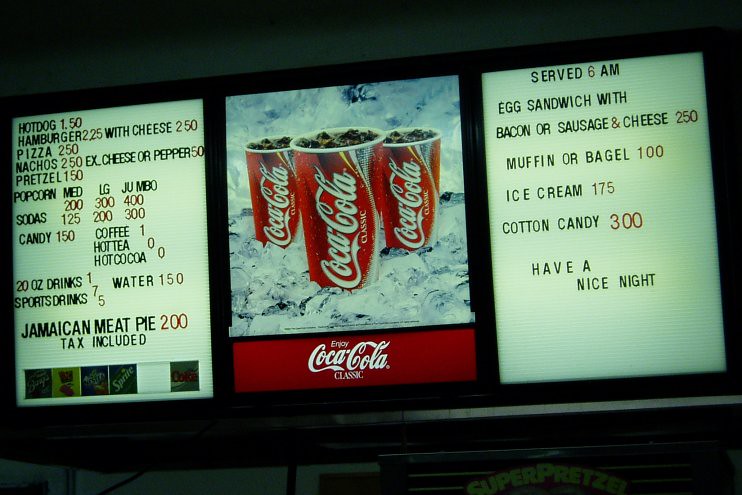The image showcases a backlit menu in a fast food restaurant. Dominating the center of the menu is a vivid square image featuring three Coca-Cola cups, filled to the brim with Coca-Cola and topped with ice. Surrounding this central image are icy visuals and glaciers, enhancing the refreshing appeal. Below this, a red rectangular sign with the classic Coca-Cola logo and the words "Coca-Cola Classic Enjoy" in white text adds a nostalgic touch.

To the left of this central image, a detailed menu lists various food items with corresponding prices in red text:
- Hot Dog: $1.50
- Hamburger: $2.25 (with Cheese: $2.50)
- Pizza: $2.50
- Nachos: $2.50
- Extra Cheese or Pepper: $0.50
- Pretzel: $1.50
- Popcorn (Medium: $2, Large: $3, Jumbo: $4)
- Sodas (Small: $1.25, Medium: $2, Large: $3, Jumbo: $3)
- Candies: $1.50
- Coffee: $1.00
- Hot Tea: $0.00
- Hot Cocoa: $0.20
- Sports Drinks: $0.75
- Water: $1.50
- Jamaican Meat Pie: $2.00

The bottom of this left-side menu features images of beverages including root beer, Hi-C, Nestea, Sprite, and Diet Coke, accompanied by a blank space for additional items.

To the right of the central Coca-Cola image, another menu section lists breakfast items, also with prices in red text:
- Egg Sandwich with Bacon or Sausage and Cheese: $2.50
- Muffin or Bagel: $1.00
- Ice Cream: $1.75
- Cotton Candy: $3.00
A friendly message "Have a nice night" is included at the bottom. All text on this section is in black, with prices distinctly highlighted in red.

Beneath the menu on the bottom right-hand corner, the top of a pretzel machine is visible, branded with "Super Pretzel" in bold yellow text at the top, adding another touch of classic snack bar charm.